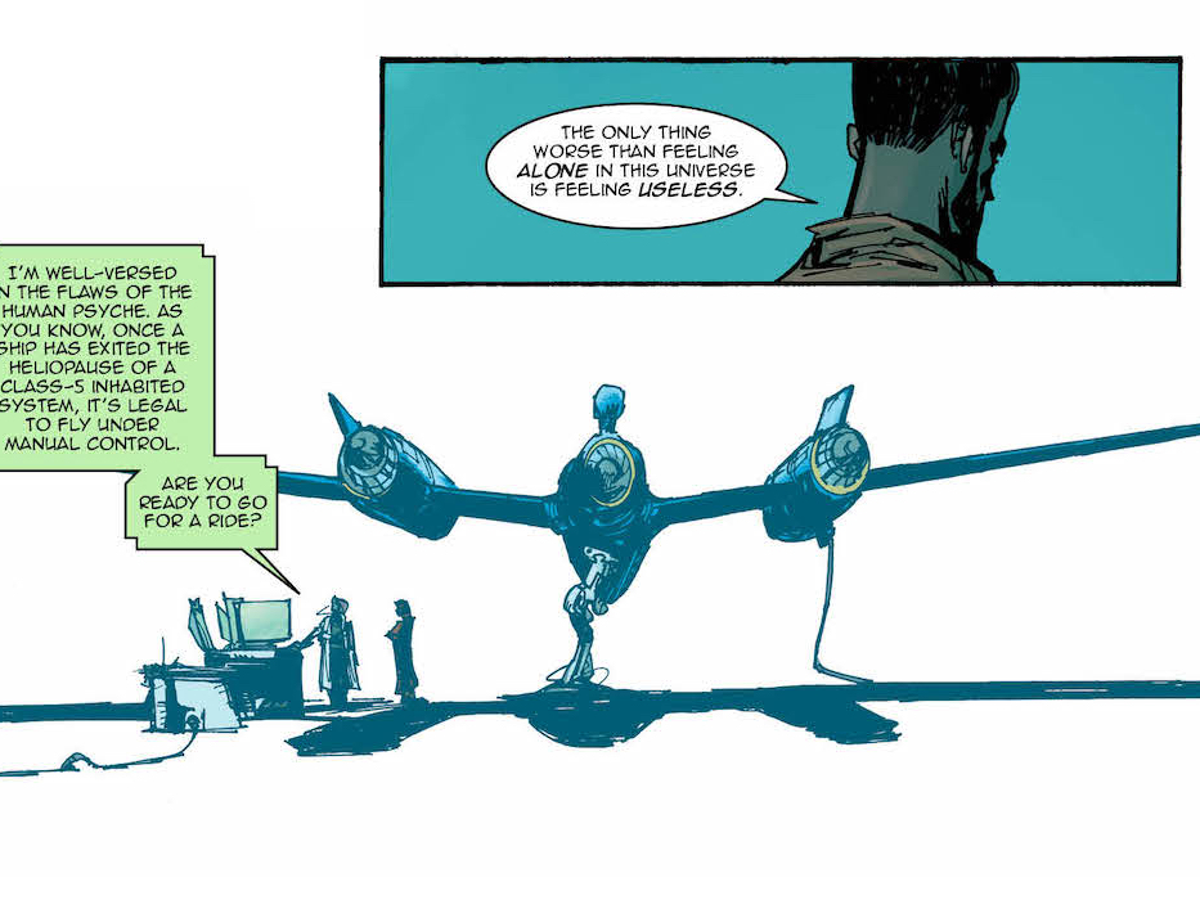This detailed comic book panel predominantly features blue hues and dark tones. The upper right-hand corner of the panel includes a rectangular inset with a blue background, showing the back of a man's head. He has short dark hair, possibly a beard, and wears gray tones. His dialogue reads, "The only thing worse than feeling alone in this universe is feeling useless."

The lower part of the panel illustrates a spacecraft that resembles a jet, entirely rendered in shades of blue, with a shadow beneath it. This spacecraft, which has two wings each with a blue cylinder attached, is situated to the right of a control desk adorned with screens and wires. Two figures, vaguely depicted in blue silhouette, are conversing beside the desk. One of them states, "I'm well-versed in the flaws of the human psyche. As you know, once a ship has exited the heliopause of a Class 5 inhabited system, it's legal to fly under manual control. Are you ready to go for a ride?" The simplicity of the background suggests an indoor setting, such as a hangar or laboratory.